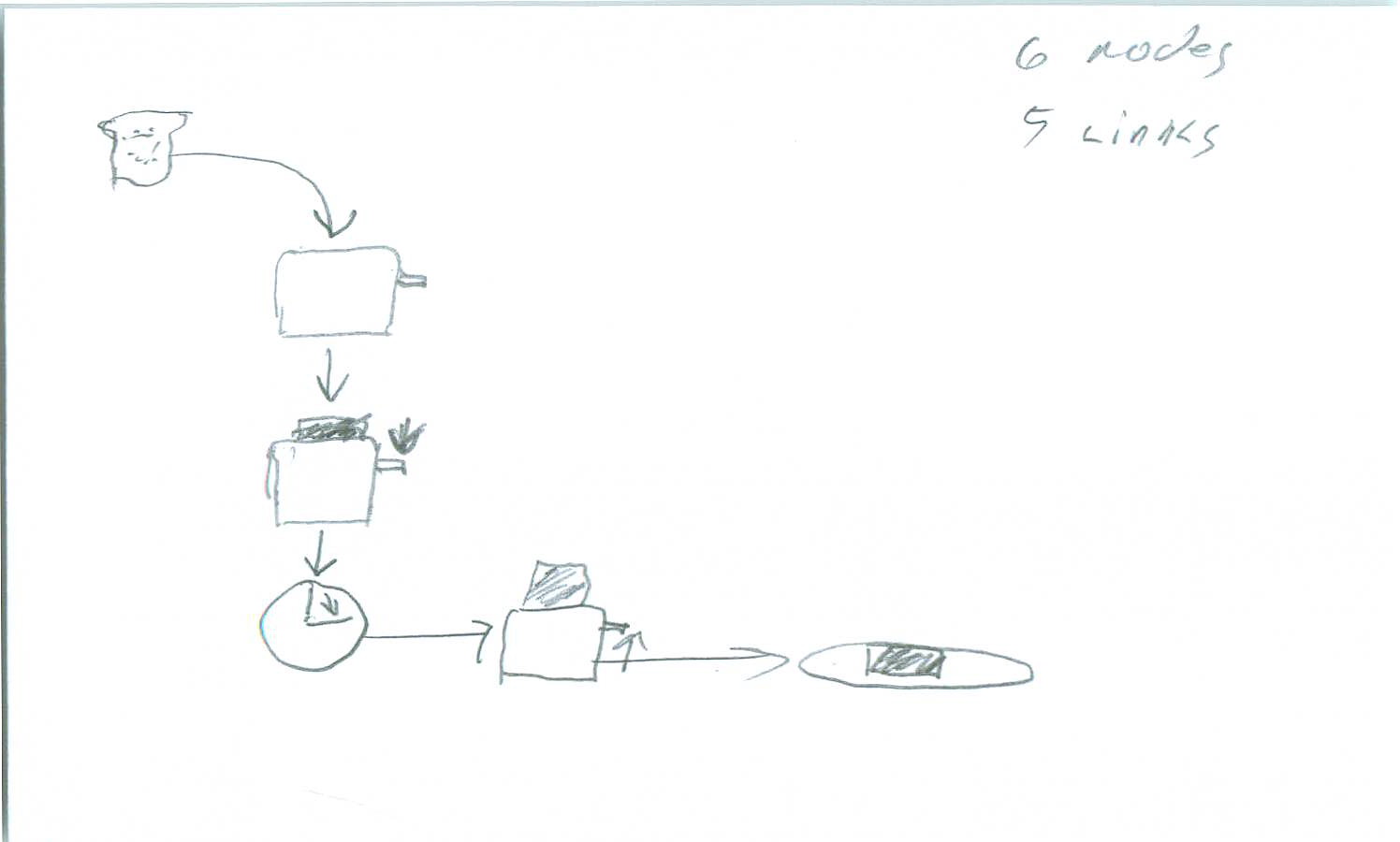This detailed pencil drawing on a white piece of paper illustrates the stages of toasting bread with clear, sequential arrows guiding the viewer through the process. At the top right corner of the paper, there is a handwritten note that reads "six nodes, five links."

On the left side of the paper, there is an initial drawing of a piece of bread, slightly curved at the top, with intricate lines and circles inside it, placed within a square outline. A curved arrow points downwards from this bread illustration to a toaster depicted below. This toaster is a square box with a handle on the right side.

Following the sequence, another downward arrow shows the bread now positioned inside the toaster. The bread is shaded dark, indicating it is in the toasting process. Nearby, an arrow points at the toaster's handle, illustrating its interaction. Below this setup, a further arrow points downward to a clock face with a wedge-shaped area, symbolizing the timing mechanism.

An arrow extends rightward from the clock to the toaster icon, showing the process after the timer is engaged. The bread inside the toaster has popped up and is noticeably darker, indicating it is toasted. An upward arrow underlines the final toast position after the handle is released.

From the right side of the toaster, another arrow points towards a subsequent drawing of a plate with the toasted bread placed on top. This final scene completes the visual narrative of the toasting process, effectively transformed from conceptual bread to a ready-to-eat piece of toast on a plate.